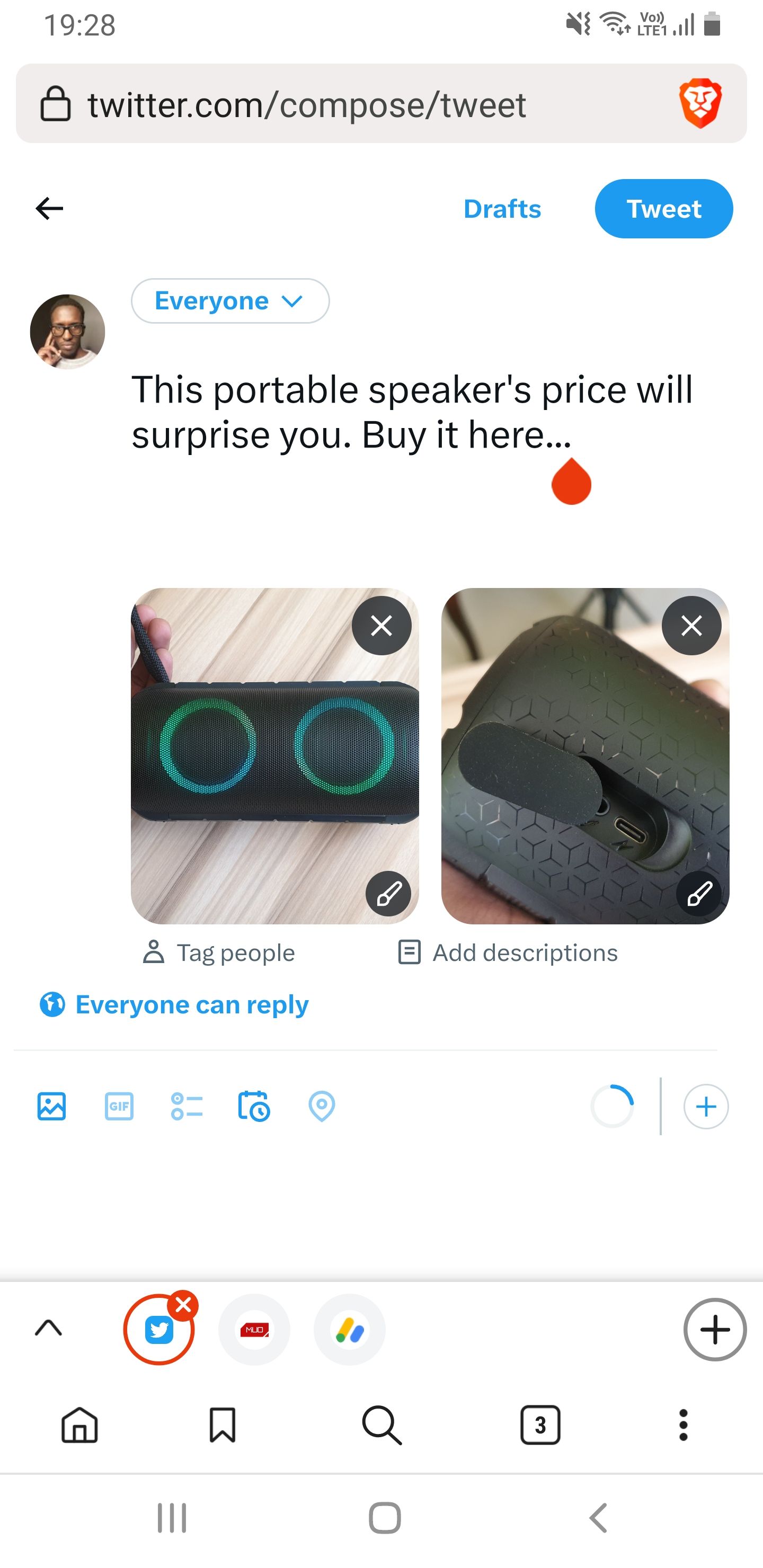The image is a screen capture taken from a mobile device, displaying a Twitter webpage. At the top, on a grey horizontal bar, there is a secure icon resembling a padlock followed by the URL "twitter.com/compose/tweet". Just below, there's a back arrow pointing to the left. The user has a round profile picture showing a person wearing glasses, located on the left side. Next to the profile picture, within a small grey-edged rectangle, the word "Everyone" is displayed in blue, indicating the tweet's visibility settings. 

Below this, a promotional tweet is written in black text: "This portable speaker's price will surprise you. Buy it here." A red drop emoji follows the text, likely for emphasis. Beneath the emoji are two images displaying different views of the portable speaker. Further down, in blue text, it is noted that "Everyone can reply," indicating the tweet's reply settings.